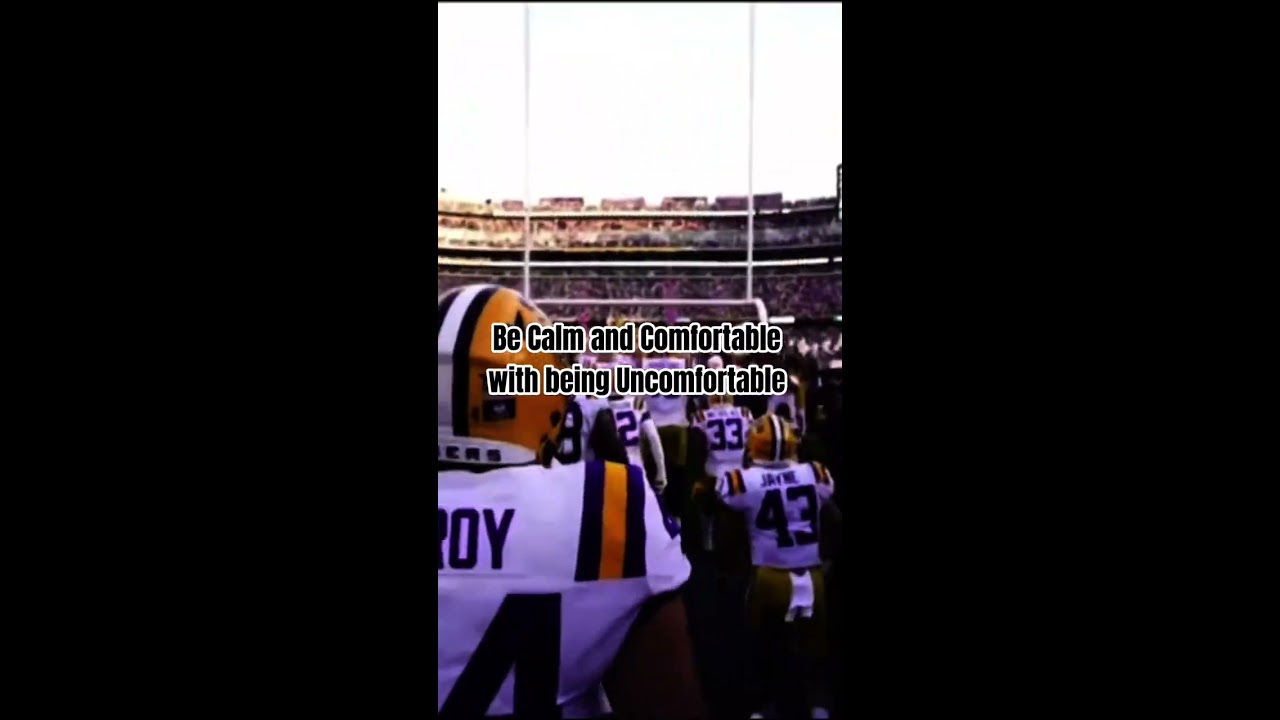The image captures a dynamic scene from an American football game set in a packed stadium. The focal point is a group of players in white jerseys with orange and blue stripes, huddled together on the green grass, moving energetically towards the goal posts visible in the background. The players wear predominantly orange helmets, each featuring a white stripe bordered by black lines. Amidst them, the numbers 33 and 43 stand out on the right-hand side, while another player partially obscures his number, showing only the top portion of a four. The scene is framed vertically, flanked by black borders on either side, giving it a retro mobile phone-like appearance. Above the bustling players and under a visibly white sky, the crowd fills the stadium, adding to the atmosphere. Superimposed across the middle of the image, bold black text with a white outline reads, "Be calm and comfortable with being uncomfortable". The slightly grainy quality of the image suggests it might hark back to an older era, perhaps giving it a nostalgic feel.